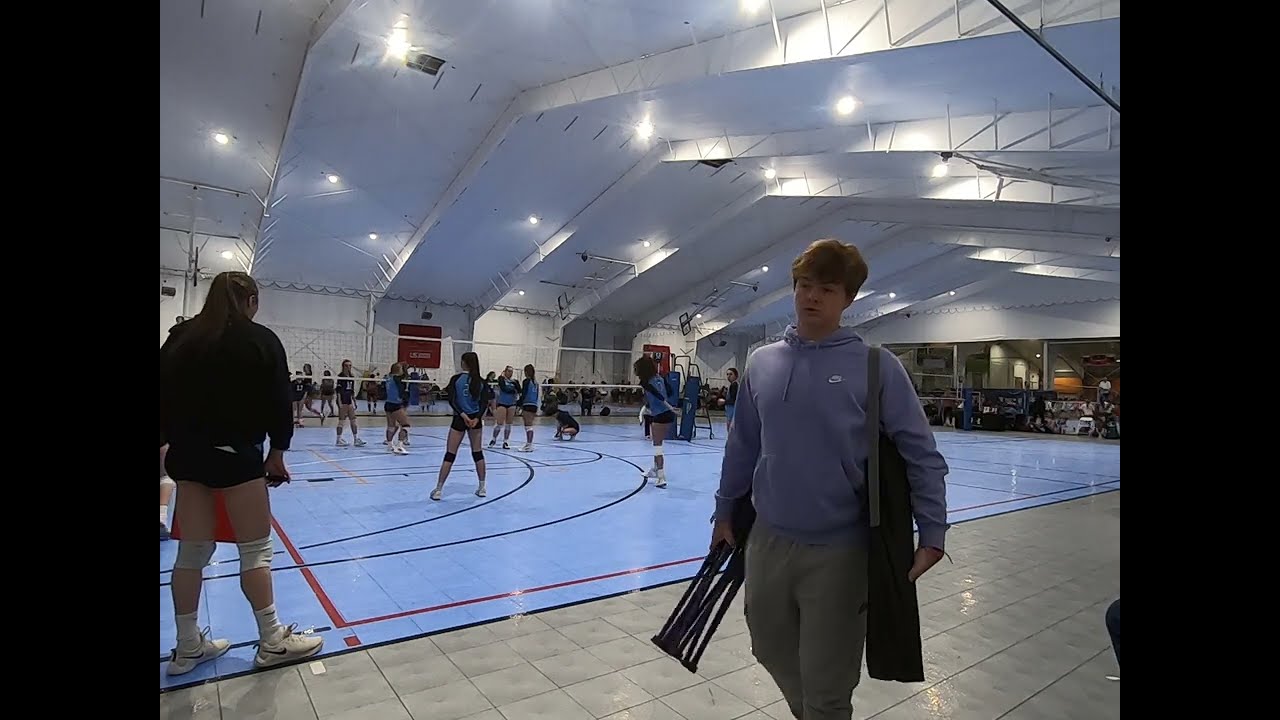The image captures the lively atmosphere of an indoor volleyball stadium, likely set in a high school. The main focus is on two volleyball teams actively engaged in their games on a baby blue court, outlined with black and red lines and bordered by gray tiles. The teams are composed of girls uniformly dressed in black shorts and blue long-sleeve jerseys, all sporting white tennis shoes. In the foreground, a young man with short dirty blonde hair walks by, dressed in a blue Nike hoodie and gray sweatpants, carrying what appears to be a tripod. The stadium's ceiling is supported by white beams, shaped into a triangular design, adorned with numerous spotlights illuminating the space. The walls are predominantly white, punctuated by red banners or possibly scoreboards, and a few windows letting in natural light. The overall scene is a vivid depiction of a bustling high school sports event.